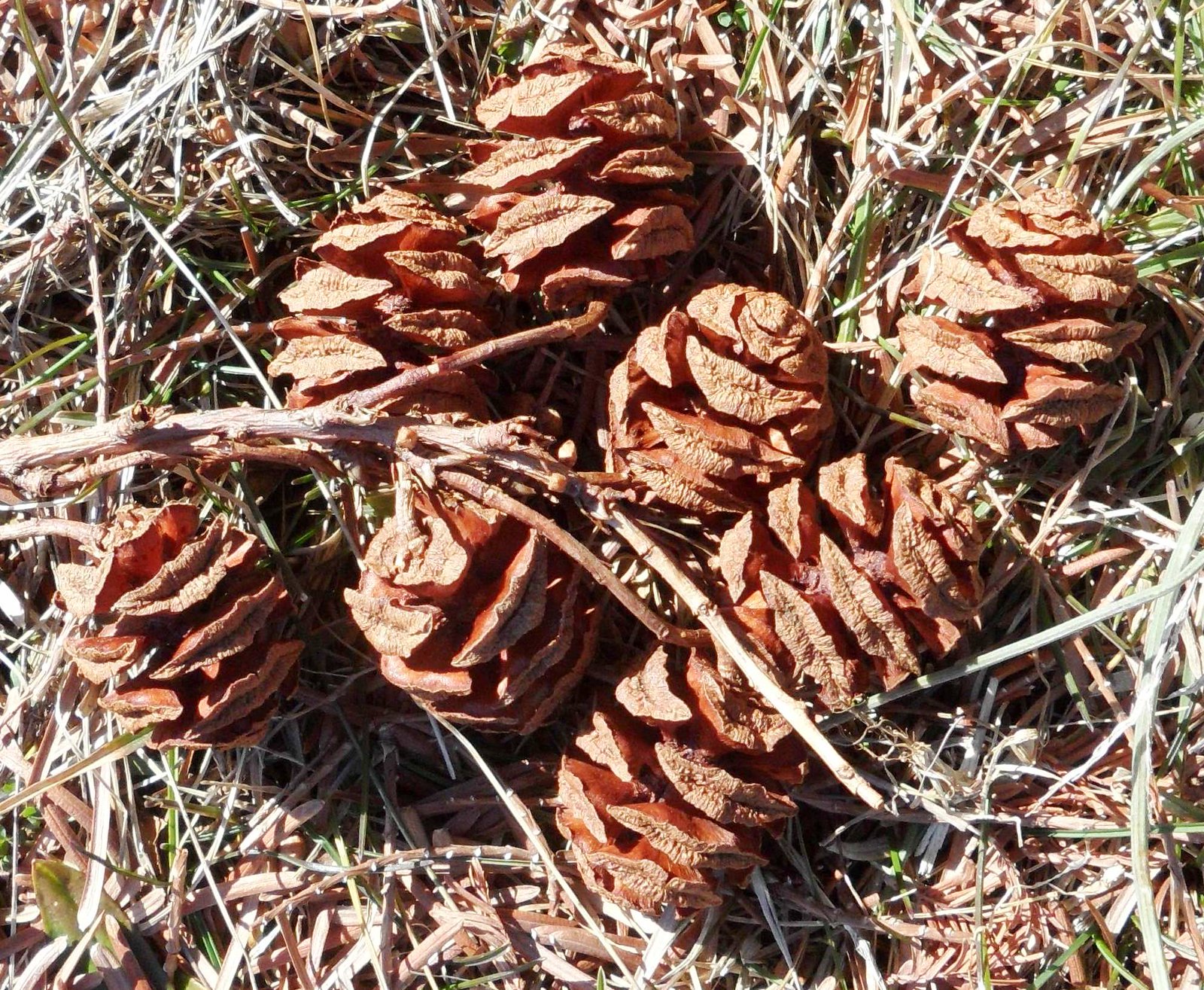The photograph or photorealistic image captures a close-up scene on a forest floor, spotlighting a group of eight uniquely shaped, orangey pinecones. These pinecones, clustered together without any particular order, exhibit a fleshy orange interior and ridged outsides that are lighter in color. The earthy background is layered with a mix of green, gold, and brown hues, composed of leaves, grass, and twigs, with a large branch diagonally draped over some of the pinecones. The scene is bathed in daylight, casting ample light on the pinecones and the surrounding debris, emphasizing their detailed textures and blending colors.